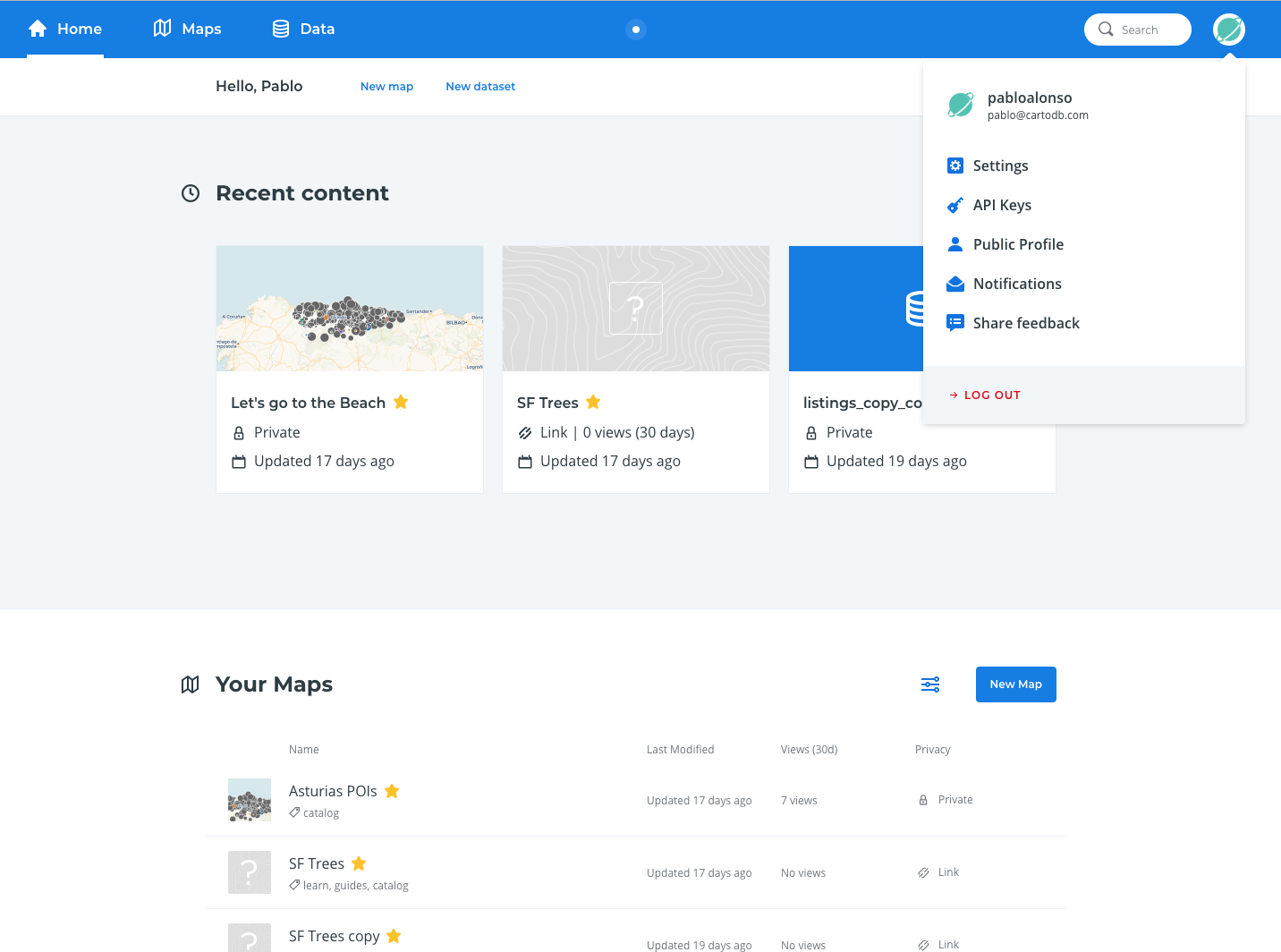The image depicts a webpage with a blue header at the top. On the top left of the header, "Home" is displayed in white text, followed by "Maps," "Data," and "Search" on the far right. There is a green planet icon, which appears to be a user photo, and it is currently selected. 

A pop-up menu is situated under this icon, displaying the username along with options such as "Settings," "API Keys," "Public Profile," "Notifications," "Share Feedback," and "Logout," the last of which is highlighted in red. Below the blue header, there is a white banner with the text "Hello Pablo" towards the left, and to its right are buttons labeled "New Map" and "New Data Set."

The main body of the webpage begins with another blue section labeled "Recent Content" at the top left, featuring three thumbnails. Below this section, the background changes to white, and on the left side, there is a category labeled "Your Maps," displaying various maps that have been selected.